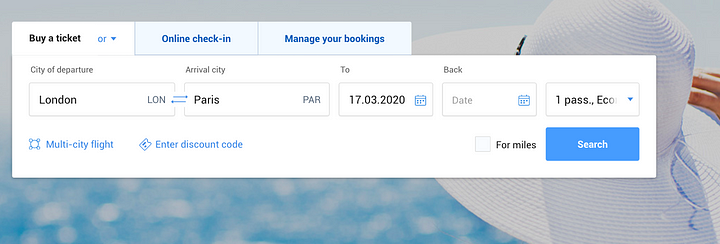The image displayed on the web page features a visually appealing backdrop and functional elements aimed at individuals arranging a flight. The photograph in the background captures an idyllic scene: the top of a woman’s head adorned with a wide-brimmed, white straw hat, shielding her from the sunny day. Her right hand rests elegantly on the brim of her hat, hinting at her relaxed demeanor. The sparkling blue waters and bright sunlight evoke a sense of travel and adventure.

Overlaying this serene imagery is a white rectangular box that houses all the essential flight information. At the top of this box are three tabs labeled "Buy a Ticket," "Online Check-in," and "Manage Your Bookings." The "Buy a Ticket" tab is highlighted in white with black text, indicating it's the currently active tab, while the other two tabs display light blue backgrounds with bright blue text.

Beneath the tabs, the interface is designed for ease of use. In gray text, the options "City of Departure" and "Arrival City" are presented horizontally across the page, followed by fields for "To" (indicating the date) and "Back" (which is currently not filled out), along with a passenger and class selector. Under "City of Departure," there is a box filled with the text "London" in black, and under "Arrival City," the box reads "Paris" in black text. The date "3-17-2020" is specified in the "To" field. The final box on the right-hand side indicates "one passenger, economy."

At the bottom of this structured layout is a bright blue search button, compellingly marked with the word "Search" in white, inviting the user to proceed with finding their flight options.